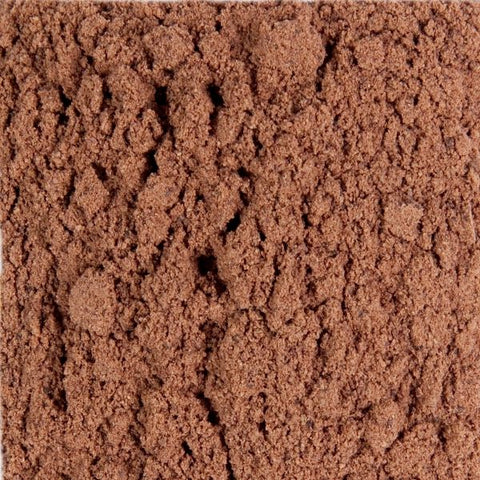This is a detailed close-up photograph of a textured, brown surface. The entire square-shaped image is dominated by this substance, which has the rich, earthy color and granular look reminiscent of cinnamon. The surface features a mixture of cracked and clumpy areas, with the most prominent cracks appearing in the middle and top-left sections of the frame, while the right side of the image has fewer cracks. The substance, likely soil or possibly a granular material like brown sugar or finely ground stone, contains dark holes and clumps formed from bunching. The image does not contain any other elements, focusing solely on this intricate and rugged texture.